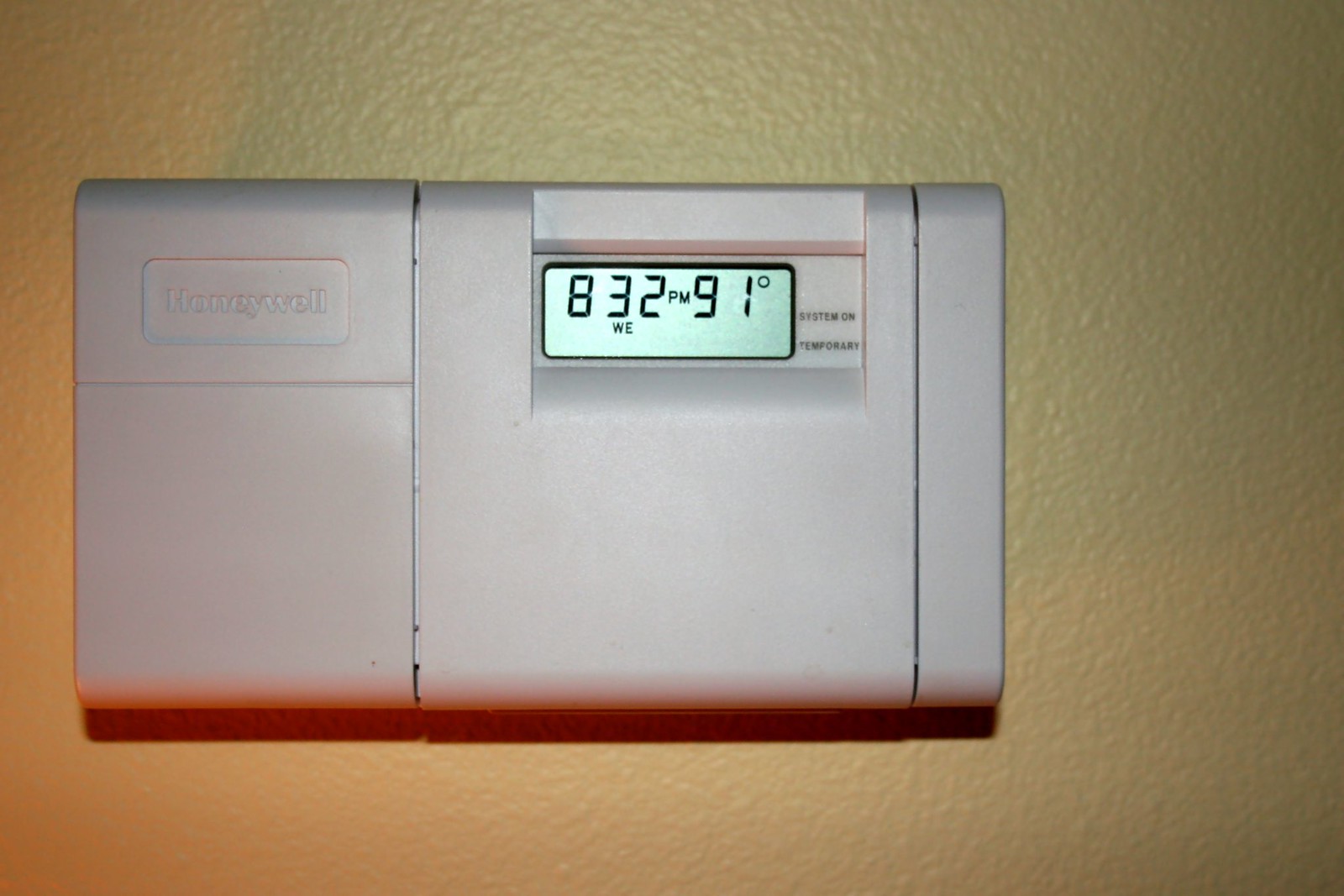In the photograph, a Honeywell thermostat is mounted on a textured tan wall, which exhibits a subtle gradient with a lighter tone in the lower left corner and a darker shade in the upper right corner. The thermostat is centrally positioned towards the left side of the image and features a predominantly solid white rectangular design. The Honeywell logo is embossed in a small rectangle located in the upper left corner of the device.

The thermostat’s display screen is situated in the upper right corner and occupies approximately 20% of the device's right side. The screen displays the current time as 8:32 PM in a machine-like font. To the immediate right of the time, the temperature reads 91 degrees, and below the number '3' are the letters 'WE'. Additionally, the word 'System' is visible on the right-hand side of the display, with a partially legible word that appears to be 'Temporary'. The overall presentation and digital readout reflect the modern and functional design characteristic of Honeywell thermostats.